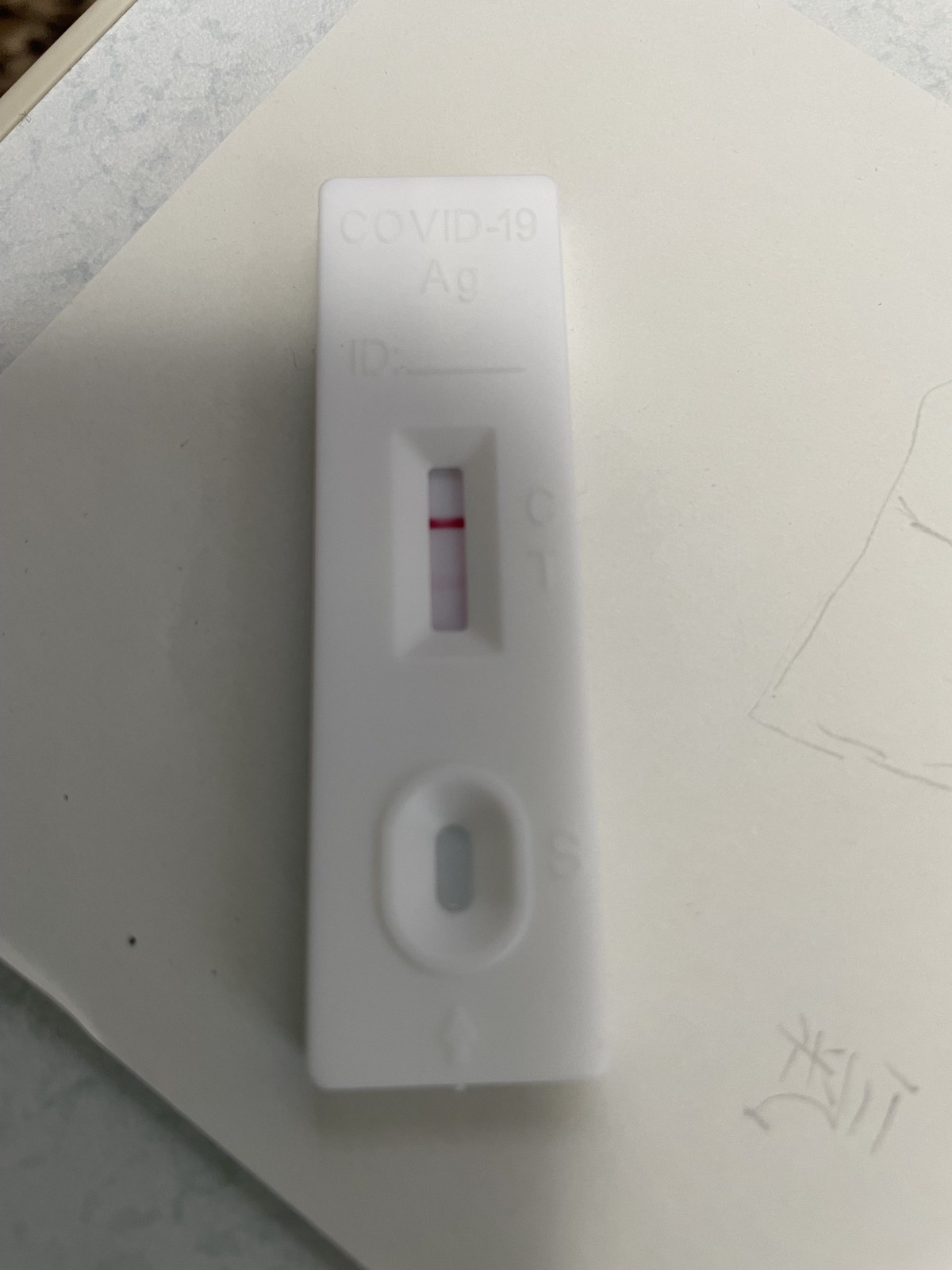The photograph captures a close-up view of a white plastic COVID-19 test placed on a countertop. The test strip features an oval area labeled 'S' to the right, with an arrow pointing towards a slit marked by the letters 'C' at the top and 'T' at the bottom. Above this slit, the label reads 'ID:' followed by an underline and 'COVID-19 AG.' The test indicates a bright red line next to 'C' and a very faint pink line next to 'T', making it unclear whether the result is positive or negative. Below the test strip, there is a piece of poster board that appears to have writing and drawings, potentially in an Asian script, though it is not easily identifiable. The drawing seems to outline a square or rectangular object in pencil. The scene suggests an environment where someone may have been engaged in documentation or analysis, with the setting being a counter with the test and board casually arranged.